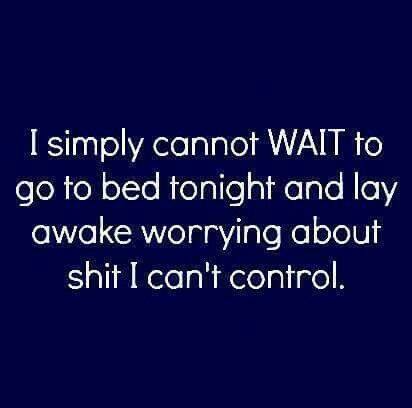"Displayed within a simple blue square, this image features the witty phrase, 'I simply cannot wait to go to bed tonight and lay awake worrying about shit I can't control,' written in white text with standard capitalization except for the word 'wait,' which is emphasized in all caps. The text is centered, with the widest spacing in the second line and the narrowest at the last, making the quote stand out clearly against the dark blue background. This humorous yet relatable statement captures a common sentiment and is the kind of meme-like image frequently shared on social media or displayed as a cheeky decoration."